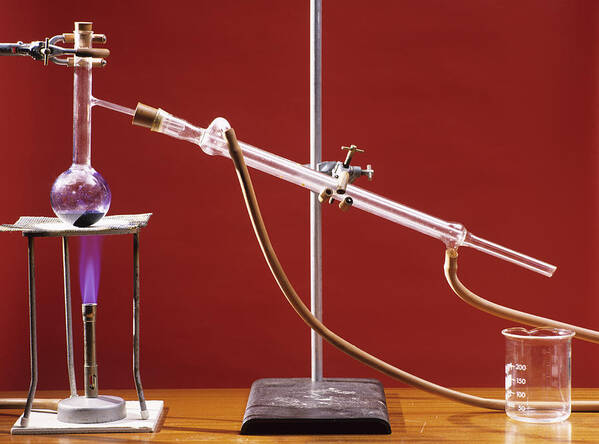The image depicts a detailed chemistry lab setup positioned on a wood-grained, light-colored countertop with a brick red wall serving as the backdrop. Central to the arrangement is a chemistry experiment involving various pieces of laboratory glassware. On the left is a clear glass beaker, while the centerpiece is a long glass test tube held by a metal stand. This test tube connects via tubing to another beaker situated above a Bunsen burner emitting a blue flame. The beaker, marked with measurement indicators from 50 to 200 milliliters, sits securely on the burner platform. Additional tubes and pipes extend from the test tube, contributing to the intricate laboratory setup without any text present in the image.